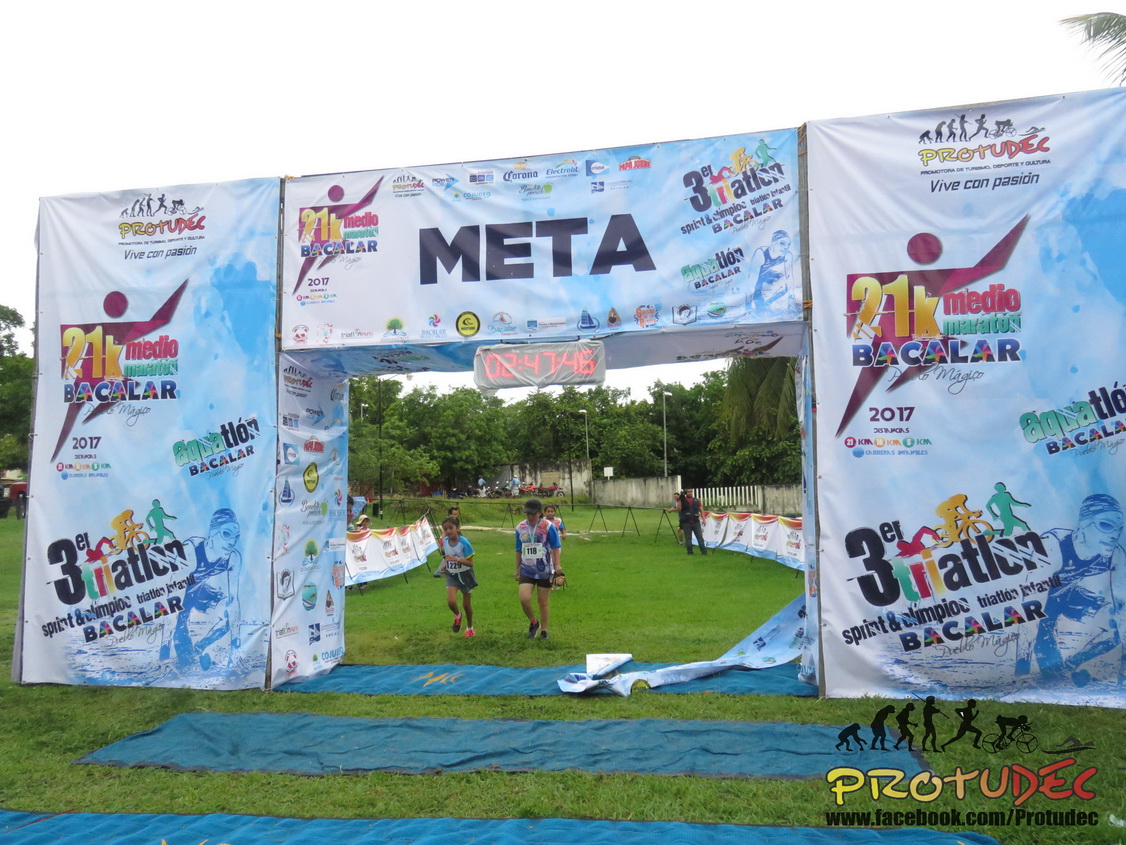The image captures a lively scene of an outdoor charity race event during the middle of the day. The setting features a grassy surface adorned with a blue canvas race lane leading up to an elaborate finish line archway. The archway is constructed of four square pillars connected by an arch that is wrapped in a tarpaulin with various graphics, primarily in Spanish. Prominent texts include "META" and "21K Media Marathon Bacalar 2017," along with sponsor logos. A time clock displayed above the runners reads 2 hours, 47 minutes, and 46 seconds.

In the center of the image, a group of runners is captured just as they cross the finish line, signifying they are not the first-place finishers as the ribbon is already broken. Among them, a young girl appears to be sprinting while an older woman beside her is walking. Both runners are dressed in blue jerseys and black shorts, wearing numbered bibs. Additional participants, including children and an individual in all black filming the event, can be seen in the background. The scene is framed by lush green grass, distant trees, and advertising banners along the race lane and on the archway. A logo at the bottom right of the image reads "prototech facebook.com." The vibrant colors of green, blue, yellow, orange, red, and white contribute to the dynamic and festive atmosphere of the race.